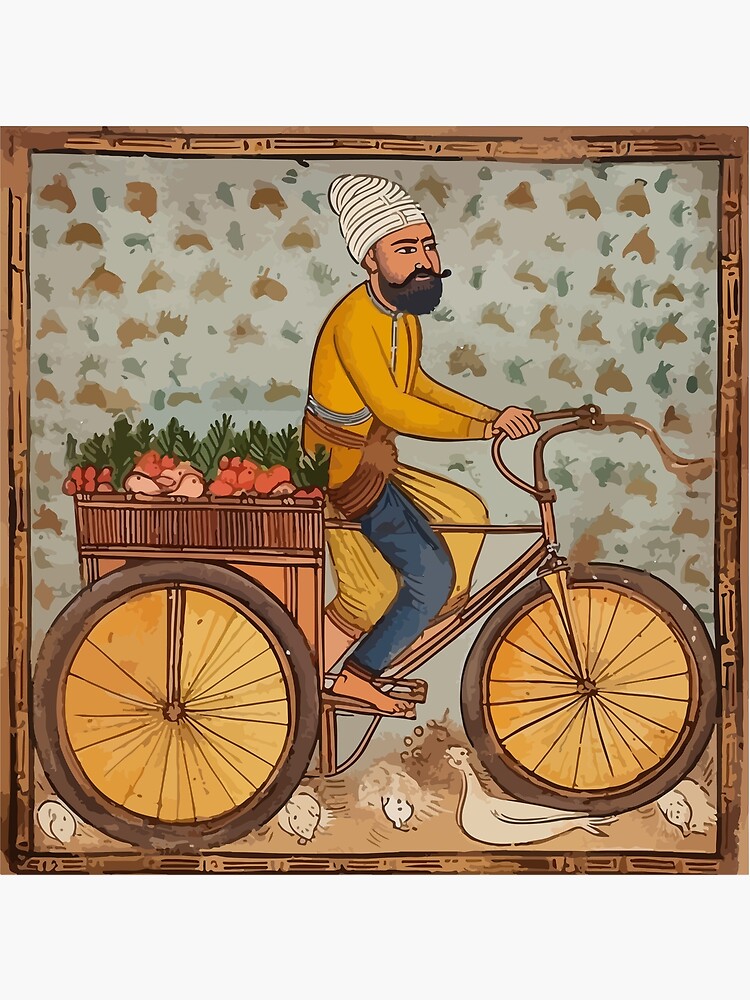The image on a white background depicts a hand-drawn scene with a brown and black geometric border. At the center, a Middle Eastern man is riding a light brown bicycle, barefoot, with a basket attached to the back. The basket is filled with red produce, possibly onions or turnips, topped with green leaves. The man, who is transporting these vegetables, is wearing a white and black headdress, a golden tunic, and navy blue trousers. He sports a full black beard and a handlebar mustache. The ground beneath the bicycle features pale birds and bits of white. The background appears to be a pattern resembling animal heads in brown on a grayish-blue surface, enhancing the image's cartoon-like, almost wallpaper-esque feel.